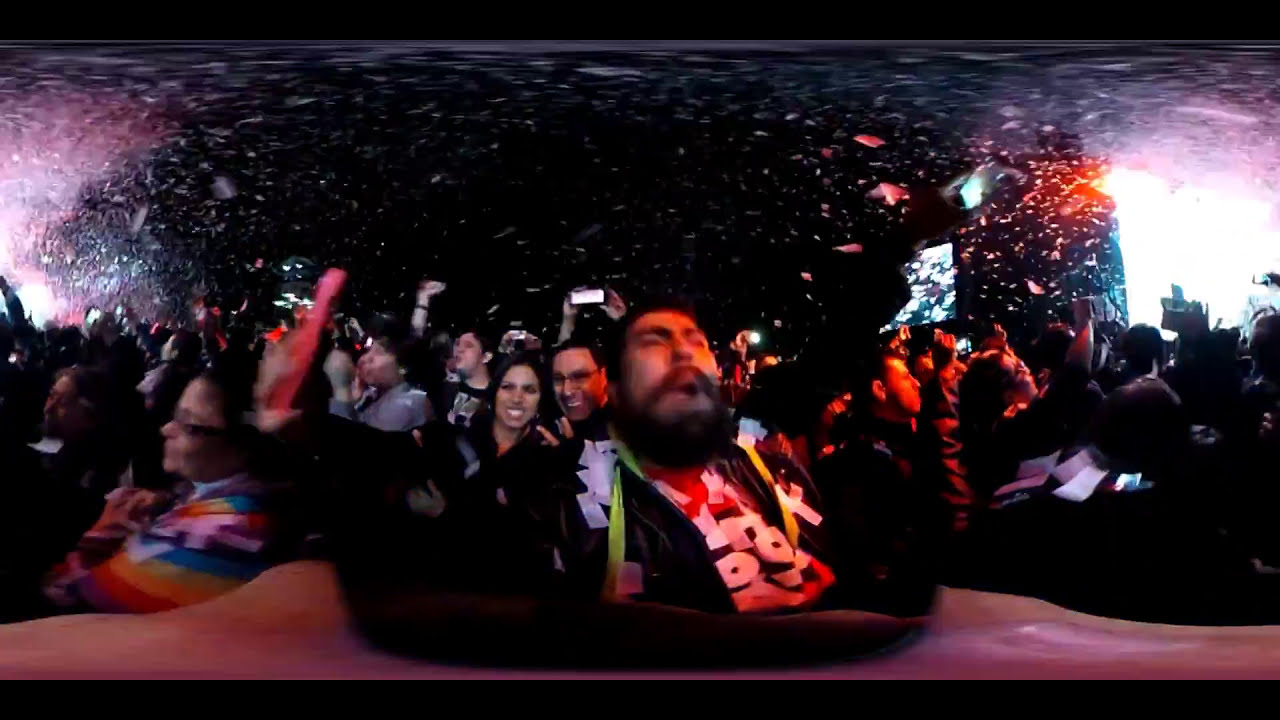In this dark and blurry photo, a large group of people is seen inside a room, seemingly attending a concert or a celebratory event. The atmosphere is electrified with excitement as confetti falls from above, adding to a festive party vibe. Bright lights in shades of red, green, orange, blue, white, and purple illuminate the background, enhancing the sense of jubilation. The crowd, a diverse array of individuals, is intently looking upwards, their faces filled with smiles and joy. At the forefront, a bearded man wearing a mix of brown, black, and red clothing stands out. He holds an object in his raised hand, his expression serious and focused. Behind him, over his left shoulder, a couple can be seen smiling. Several attendees sport colorful attire, including a person on the left in a rainbow shirt and another with yellow straps on a black jacket with a reddish shirt underneath, both looking upwards. Despite the darkness obscuring some details, the scene clearly captures a moment of shared celebration and happiness.